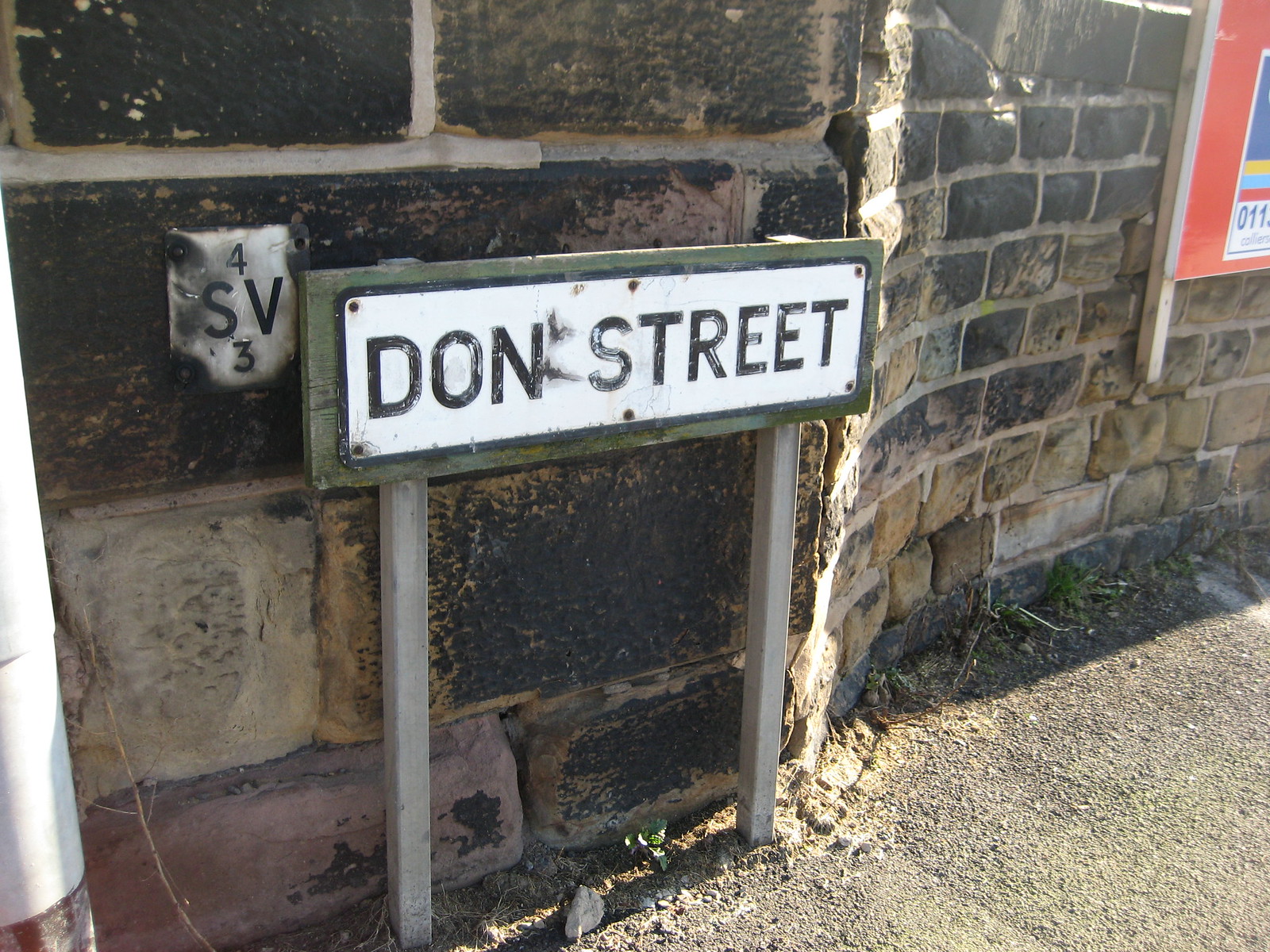The photograph captures an outdoor, midday scene centered around a weathered old stone wall composed of large, rectangular stones in varying shades of brown, black, and gold. The thick mortar between the stones looks recently refurbished in spots, adding to the aged yet maintained appearance of the wall. At the base of the image, there is a gray gravel road interspersed with patches of grass and plants. Dominating the center of the photograph is a white metal sign with a black border mounted on two metal posts. The sign prominently reads "Don Street" in black lettering. The light casts a noticeable difference in brightness on the wall, with the left side appearing darker than the right. In the top right corner, there’s another image partially visible, cut off in the background. The photograph, rectangular in shape and slightly wider than it is tall, showcases a rich palette of colors including gray, white, tan, purple, green, black, red, blue, yellow, and light blue. The setting appears to be against the wall of a historic building.